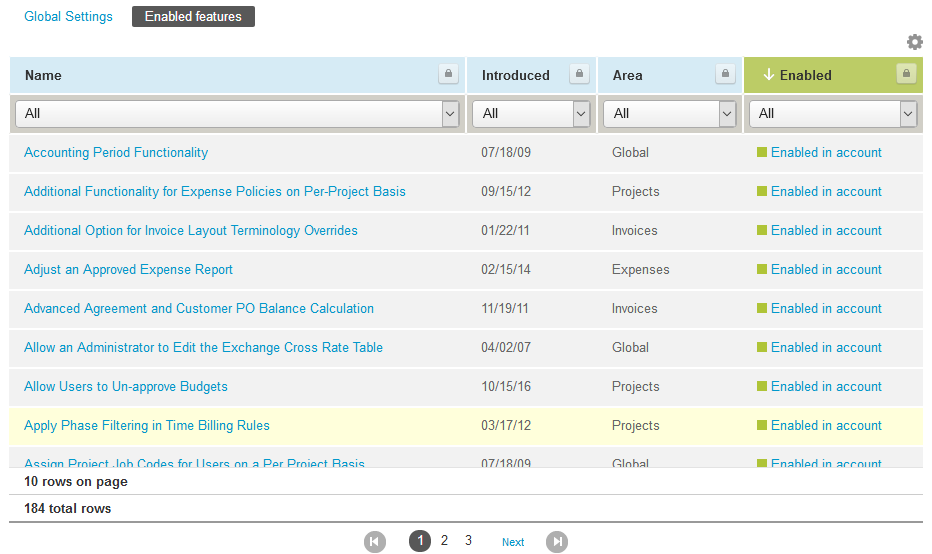The image is a screenshot of a settings interface featuring a map and various elements associated with configuration options. At the top left corner, the text "Global Settings" is prominently displayed. Directly to the right of this, "Enabled Features" is indicated, followed by a blank space, leading to a gear icon situated at the far right.

Below this top section, there is a chart with four distinct columns labeled as follows: "Name," "Introduced," "Area," and "Enabled." Each column title is accompanied by an input box with a drop-down arrow for filtering or selecting options. The first entry in this chart lists "Account Period Functionality" under the "Name" column. The "Area" column for this entry specifies it as "Global," and it is marked as enabled.